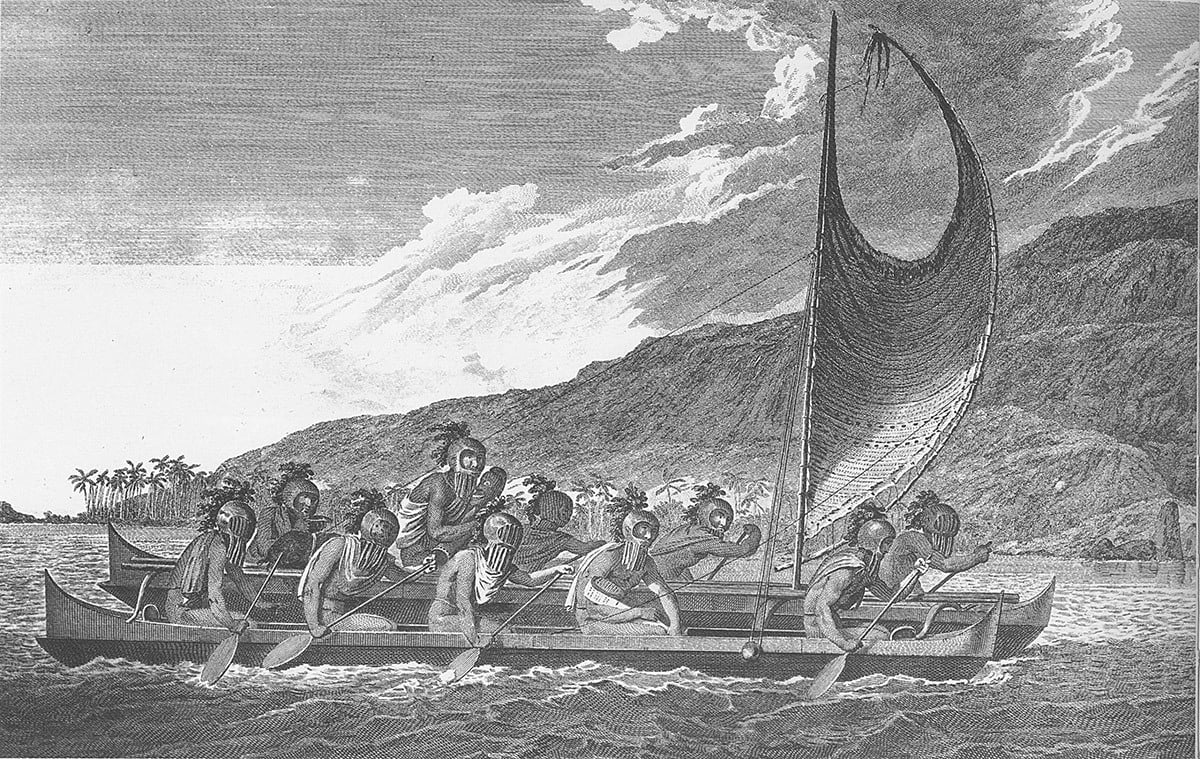This black and white historical illustration depicts a group of indigenous or potentially Polynesian people in two rowboats, each bearing a single sail. The boats, featuring ten rowers in total—with five rowers on each side of each boat—are gliding through the water towards a landmark that may be a small island. The rowers are adorned with helmets and capes, reminiscent of ancient or pagan warrior attire. In the background, a vast sky with clouds looms over the scene, and a massive mountain rises on the left side, partly surrounded by long trees. This detailed artwork, likely from the colonization period, is rendered in gray-scale tones and has the appearance of a historical illustration one might find in a history book, emphasizing both the natural setting and the traditional gear of the people.